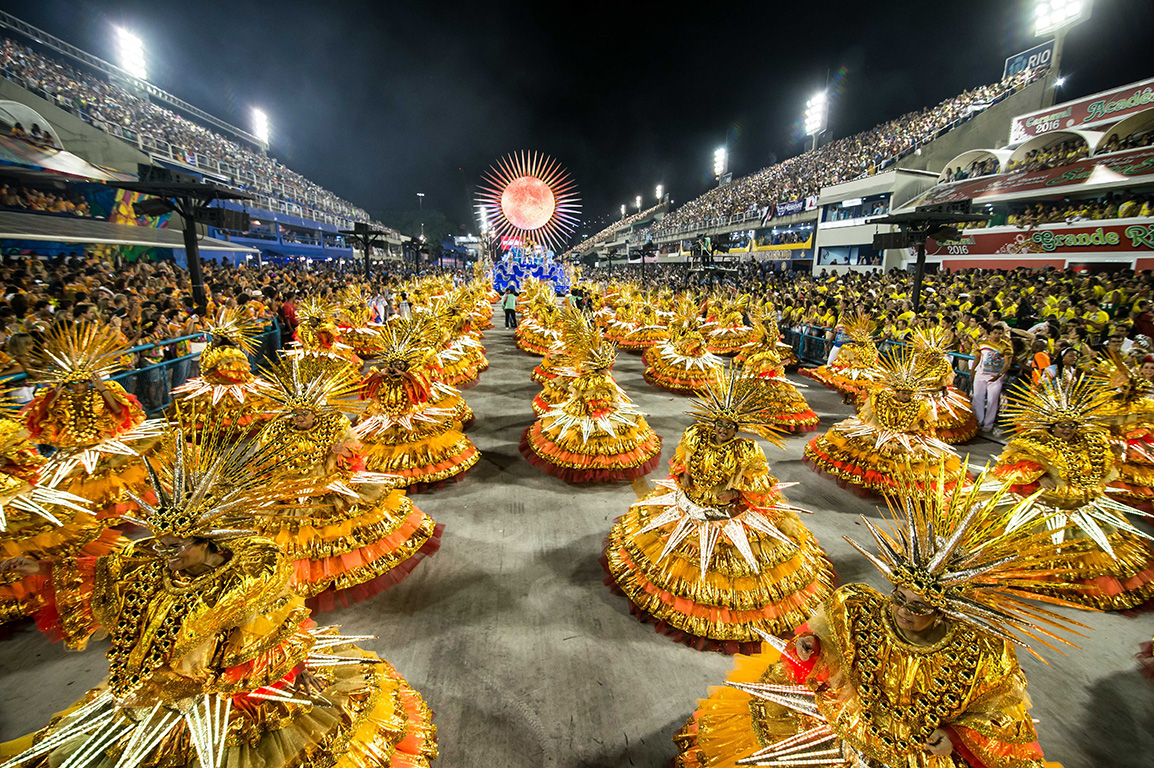The image beautifully captures a vibrant nighttime parade held in a stadium filled with thousands of spectators. Unlike a typical football stadium, this one appears narrower, with the dark night sky illuminated by stadium lights on the left and right sides. In the background, a large, glowing orange moon or sun-like sculpture radiates light beams in all directions.

Marching in the parade are rows of performers, all dressed in strikingly colorful, layered outfits predominantly in shades of gold, orange, and deeper gold. Their voluminous skirts are adorned with bright ruffles and fringe on each layer, creating a dazzling spectacle. Each performer wears an apron shaped like a white star and a significant silver, gold, and black headdress with spiky protrusions, possibly made of plastic or metal, adding to their imposing appearance. Their dark skin contrasts beautifully with their vivid attire.

The concrete-looking performance area where these women parade is surrounded by packed stands, indicating the event's popularity and grandeur. The image conveys the energy, color, and cultural richness of this captivating festival.